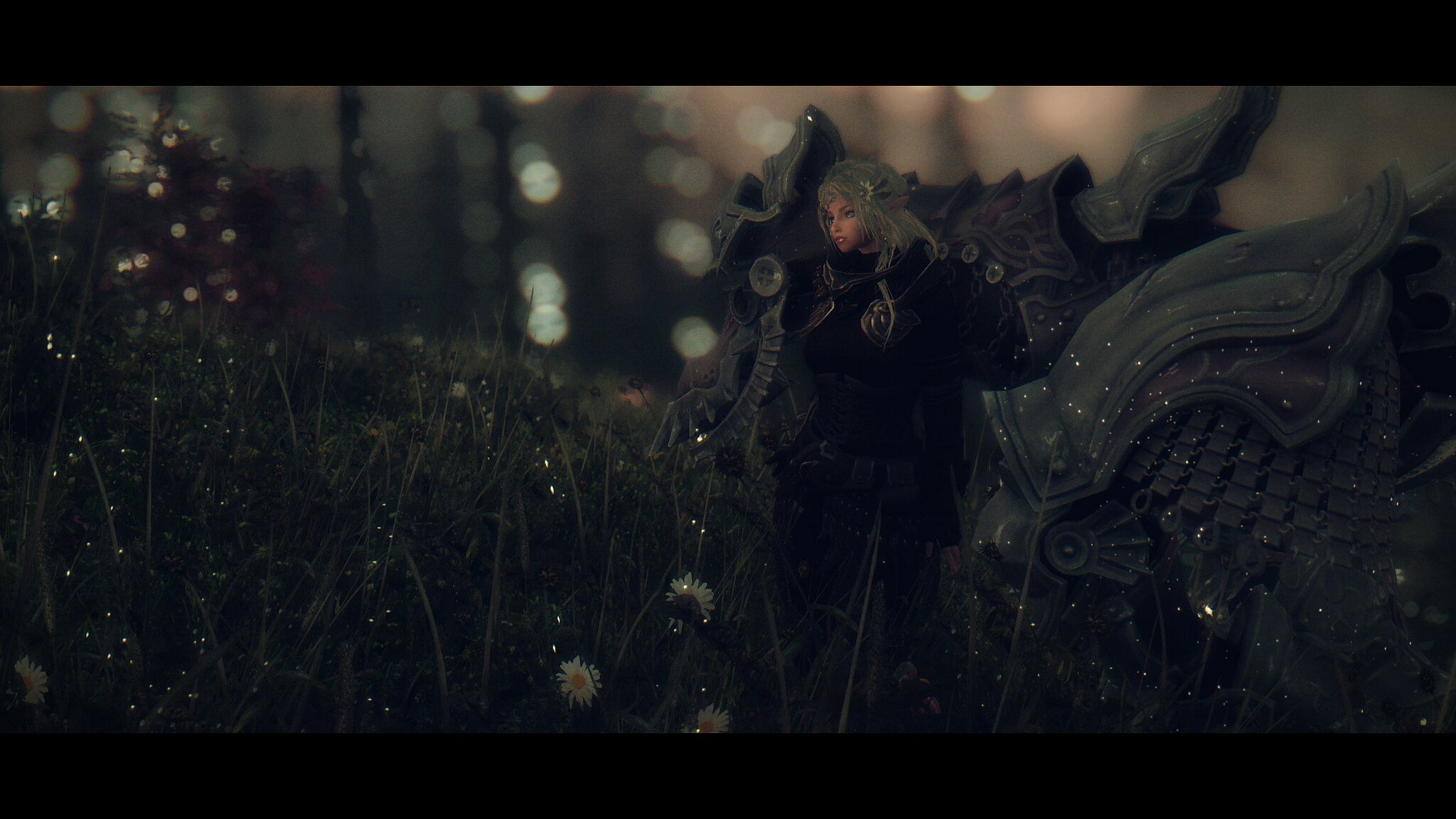This dark, atmospheric image resembles a highly detailed photograph or an artsy illustration of a regal, medieval figure. The woman at the center has long, flowing blonde hair, akin to the character from House of the Dragon, and wears an ornate black robe or possibly armor, exuding an air of nobility. Her face glows softly under a spotlight, highlighting her blue eyes and a striking yellow flower tucked in her hair, giving her an ethereal presence.

Behind her, there is a dimly lit background that suggests the etchings of a castle on one side and lush trees and greenery on the other, enhancing the mystical and enchanting feel of the scene. Adding to the fantasy, the woman appears to have either intricately designed wings or extensions of her armor made of metal or stone. The surroundings include tall, blurred grass and dandelions, with a few daisies in the foreground, and a touch of sparkle on the armor that mimics fireflies dancing around her, creating a magical ambiance. There are also mysterious, robotic lions or creatures by her side, adding an element of intrigue to the composition.